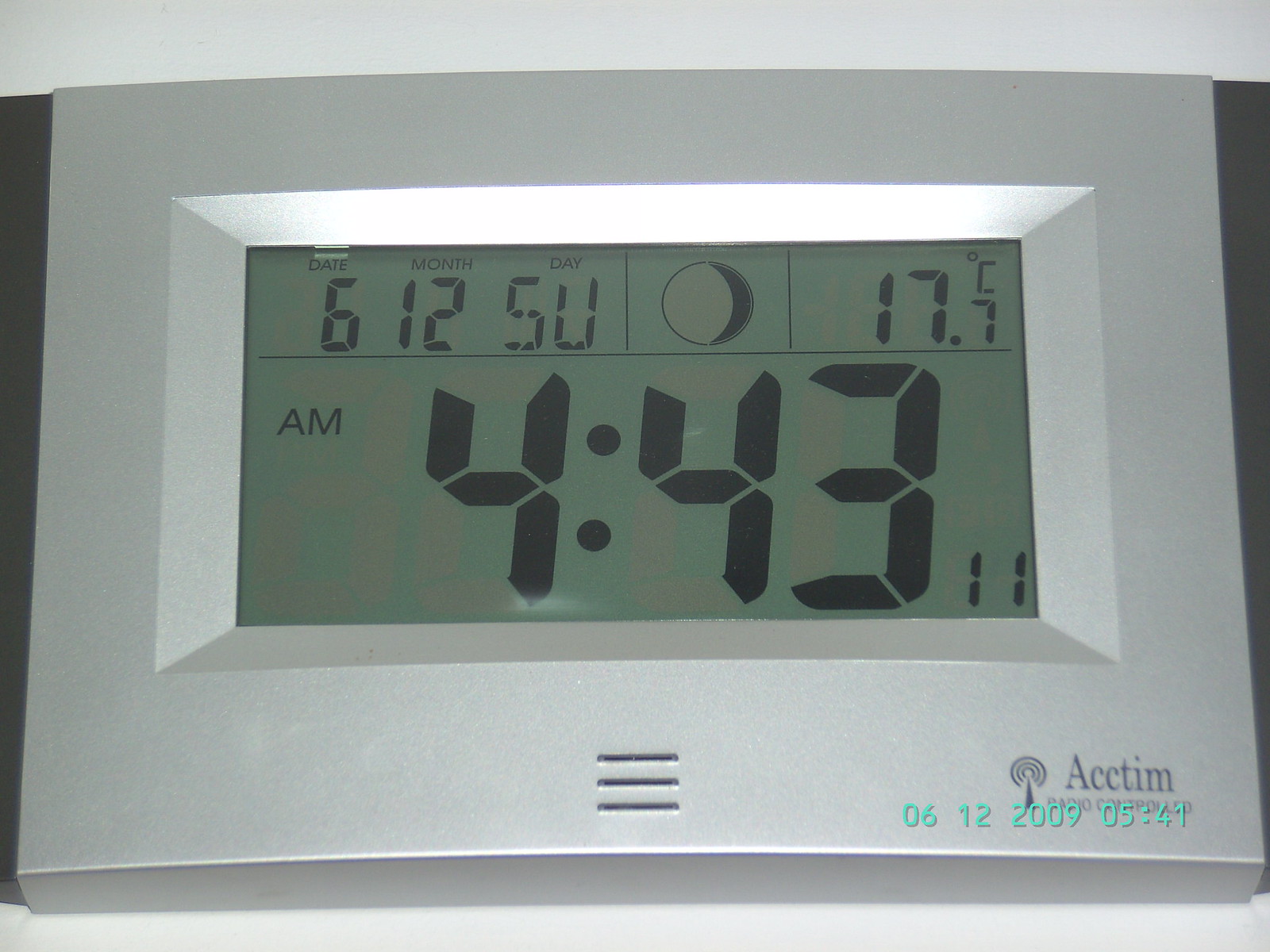A detailed descriptive caption for the photograph:

This image showcases a sleek, silver-framed electronic display, confirmed to be a radio-controlled device branded "Acctim," as noted in the bottom right corner. The display, measuring approximately 5 inches by 8 inches, features a digital interface segmented into distinct sections. At the top, it indicates the date, showing the number 6 for the day, 12 for the month, and 'SU' for Sunday. Adjacent to this is a lunar phase icon illustrating a crescent moon. The temperature is prominently displayed, reading 17.7 degrees Celsius. Dominating the bottom portion of the device are the time and additional information: the time displayed as 4:43 AM, with a small '11' positioned to the right. Overall, this device elegantly combines the functionality of showing the current date, time, temperature, and moon phase in one compact and structured format.